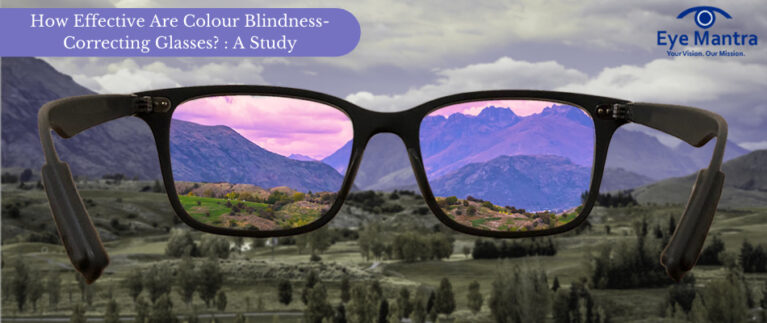The advertisement features a photograph of a picturesque mountain range with a scattering of trees on the ground and a sky filled with muted clouds. Dominating the image is a pair of black-framed glasses, positioned as if seen through the eyes of the viewer. The scene outside the lenses remains subdued and monochromatic, while the view through the lenses is vividly transformed, displaying a burst of vibrant and lively colors. 

In the upper right corner, a blue logo reads, "Imantra - Your Vision, Our Mission." Meanwhile, the upper left corner is adorned with a blue-purple stripe, containing white text that proclaims, "How Effective Are Our Colorblindness Correcting Glasses: A Study." The contrast between the dull outer world and the vibrant scene through the glasses visually emphasizes the effectiveness of the product in enhancing colors for those with color blindness.